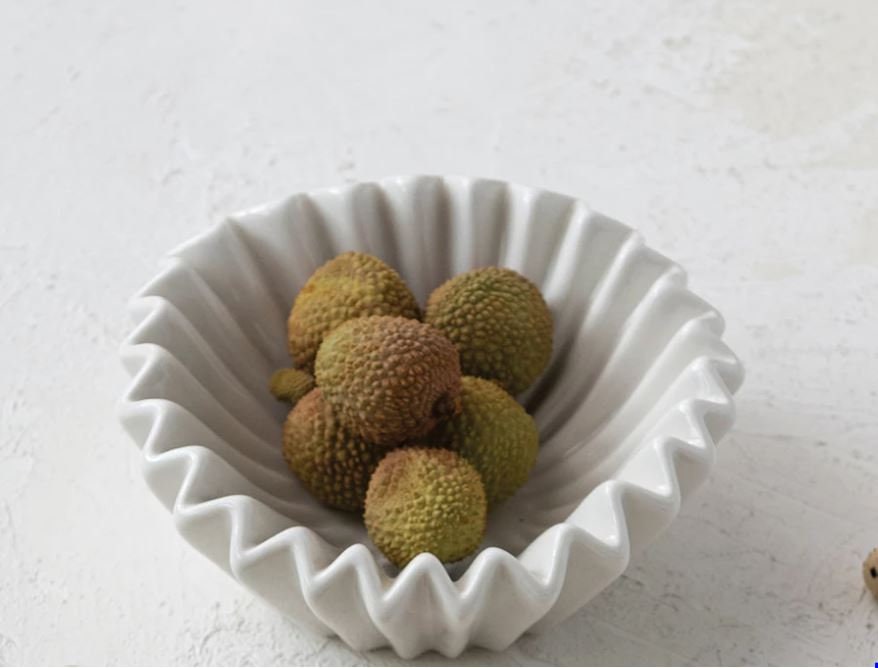This detailed photograph depicts six small lychee fruits, characterized by their green and reddish unripe skins, nestled in a thick, white ceramic bowl designed to resemble a coffee filter with corrugated sides. The bowl sits centrally on a textured, white surface that could be a counter or table. The lychee fruits are arranged with three on the right, two on the left, and one atop the others, forming a pyramid-like structure. Additionally, a seventh lychee appears to be in the background. In the bottom right corner of the image, there is a small, yellow-orange object with a black dot that vaguely resembles a mouse face seen in profile.